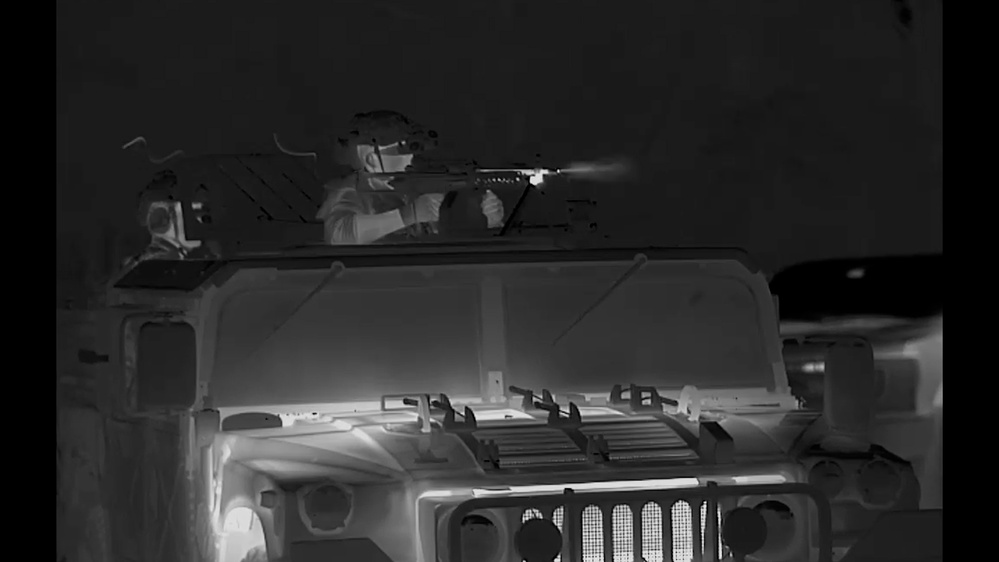The image is a detailed, black-and-white infrared night vision photograph depicting the front of a large army Humvee. The photo captures the vehicle, clearly showing its headlights and windshield. Positioned atop the Humvee, standing through a roof hatch, is a U.S. soldier identifiable by his sergeant uniform, hard hat, and night-vision goggles. He is actively firing an M16 rifle, with visible heat or flame emanating from the barrel, indicating the rifle is in use. The infrared lens also highlights the heat signatures from the soldier's skin and the engine of the Humvee. To the right of this soldier, there's the vague outline of another individual, possibly also a soldier equipped with night-vision goggles, but lacking any discernible weapon details. Another large army vehicle appears in the background to the right, adding depth to the composition.